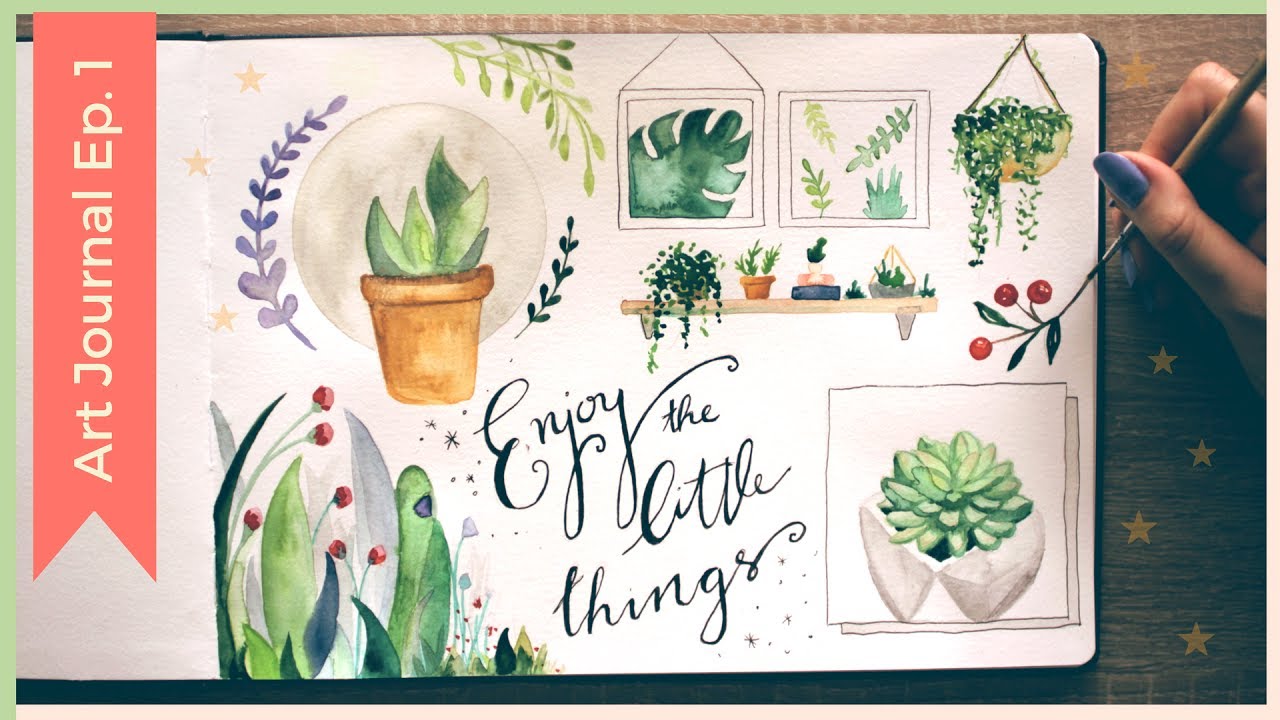In this detailed photograph, we see a young lady deeply engrossed in her arts and crafts, specifically working on her art journal. The journal prominently features the text "Art Journal, Episode One" vertically on a hanging banner. The open page she's working on is adorned with the inspiring phrase, "Enjoy the Little Things" written in cursive at the center-bottom. 

The art page is rich with botanical themes: there's a charming potted plant in the upper left corner, encircled by intricate vines, leaves, and flowers. This plant is highlighted by three yellow stars and a moon in the background. Below this, at the bottom-left corner, is a vibrant drawing of a plant with red and purple flowers. On the opposite side, the bottom-right corner hosts a soft cactus in a pot.

Her hand is captured in the act of meticulously painting a cherry blossom on the edge of the page, adding to the lush greenery theme. Above, two paintings featuring leafy designs hang against a backdrop that hints at an earthy, brown tone. Additionally, a nearby shelf supports various plant pots, including a hanging bowl of vines, a vine, a small shrub, a figure of a little man with a black hat, and a diamond-shaped statue. This image appears to be part of a tutorial series on art journaling, as suggested by the title "Art Journal, Episode One." The scene beautifully blends creativity and tranquility, showcasing the joy found in the little artistic details.